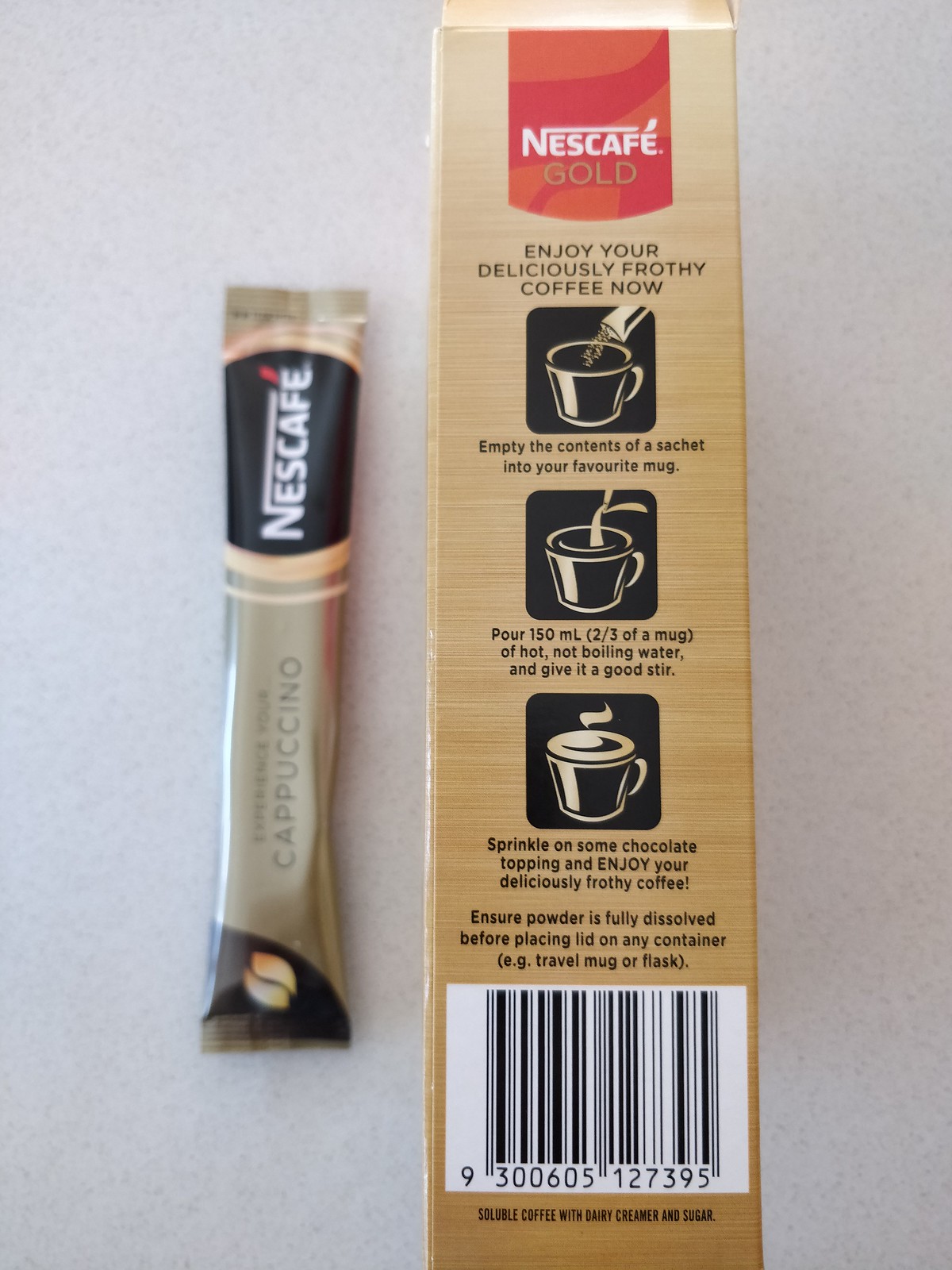This color photograph features a Nescafe Gold cappuccino box accompanied by a single-serving packet, all set against a clean white background. The attractively designed box, predominantly gold in color, showcases detailed preparation instructions on its side alongside a visible UPC code (9300605127395) at the bottom. 

The text on the box reads: "Nescafe Gold. Enjoy your deliciously frothy coffee now." Below this, step-by-step instructions are illustrated and described. These steps include: emptying the packet into your favorite mug, pouring 150 milliliters, or two-thirds of a mug, of hot (but not boiling) water, giving it a good stir, and then sprinkling some chocolate topping. It is advised to ensure the powder is fully dissolved before placing a lid on your container, like a travel mug or flask. The box further states in tiny writing that the product is "soluble coffee with dairy creamer and sugar."

The accompanying gold packet, notable for its black accents and depicted coffee bean on the far left corner, prominently displays "Nescafe" in a black circle and the word "cappuccino." The packet design complements the box, making it clear that it is part of the same premium Nescafe Gold line.